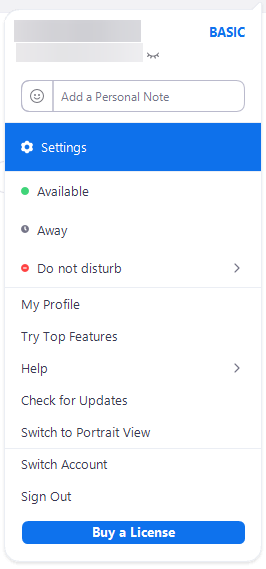The image showcases a user interface of an application featuring a clean, white background. In the top-right corner, the word "Basic" is displayed in blue text, likely indicating the app's name or version. Below, there is an input field labeled "Add a Personal Note," allowing users to type a personalized message. Below the input field are several settings buttons organized in a vertical list.

The buttons include status options such as "Available," "Away," and "Do Not Disturb," the latter having an arrow, possibly indicating a dropdown menu with additional options. Further down, the list includes options like "My Profile," "Try Top Features," and "Help," with "Help" also having a link arrow, suggesting it leads to further resources. 

Near the bottom are additional functional buttons: "Check for Updates," "Switch to Portrait View," "Switch Account," and "Sign Out." The very bottom of the interface features a prominent blue button with white text that reads "Buy a License," suggesting an option for upgrading the app or purchasing additional features.